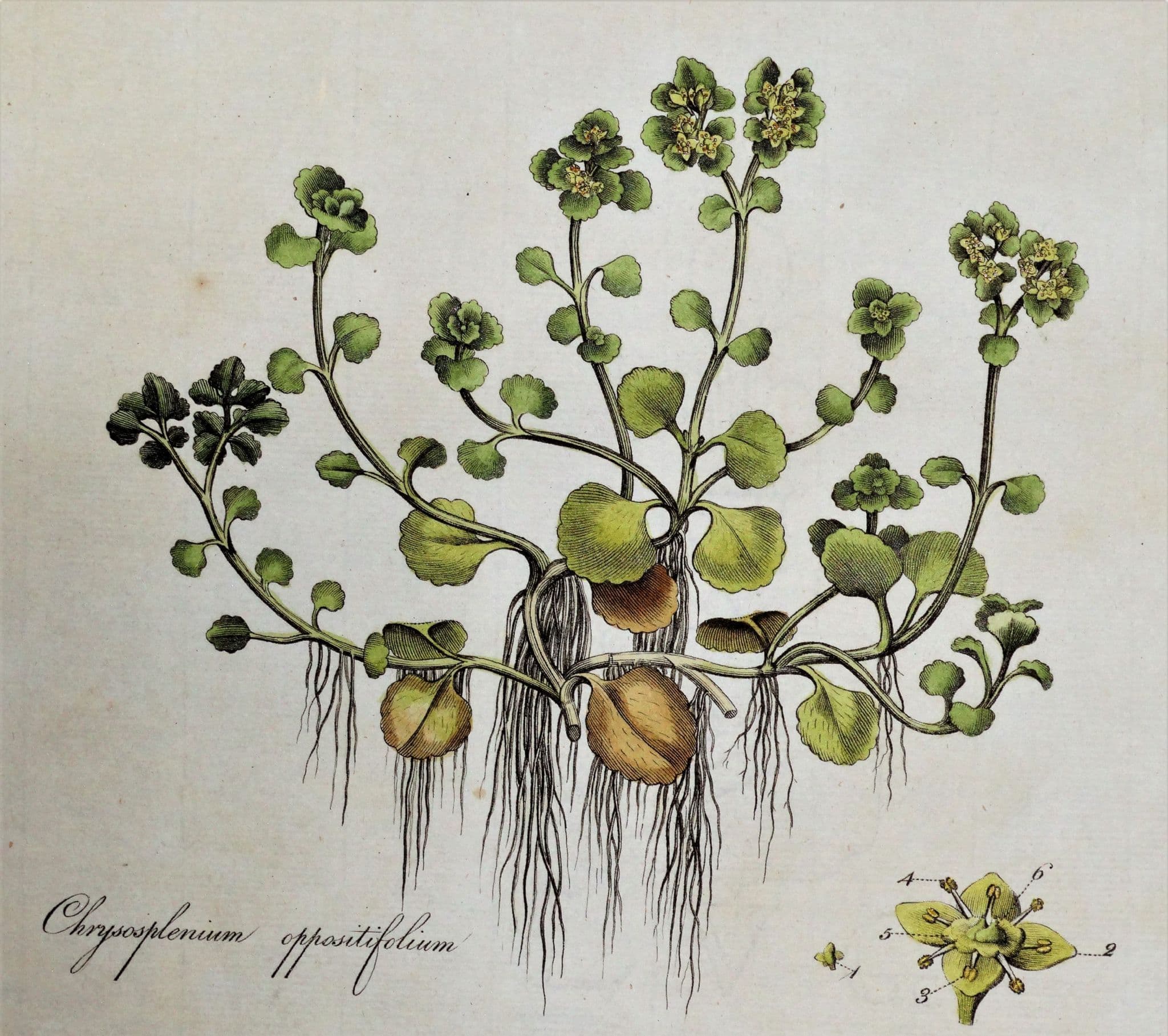The image is a detailed illustration of a plant, resembling an excerpt from a botanical book. Set against a whitish-gray background, it likely uses watercolor or colored pencil techniques. The left side of the image features elegant calligraphy, possibly in Latin, denoting the plant's scientific name, which resembles "chrysophyllinium apostifolium." The drawing shows the plant's full form, with its roots splayed at the bottom and several stems—ranging from five to nine—rising upward. These stems are adorned with clusters of green leaves and a few small yellow flowers at their tips. A close-up schematic of the flower, complete with numbered arrows for labeling, is positioned on the bottom right. While the purpose of these numbers remains unclear, no other descriptive text accompanies the image to clarify their meaning. The illustration captures the intricate details of the plant's structure, including brown leaves at the base and the complex arrangement of its leafy stems and flowers.